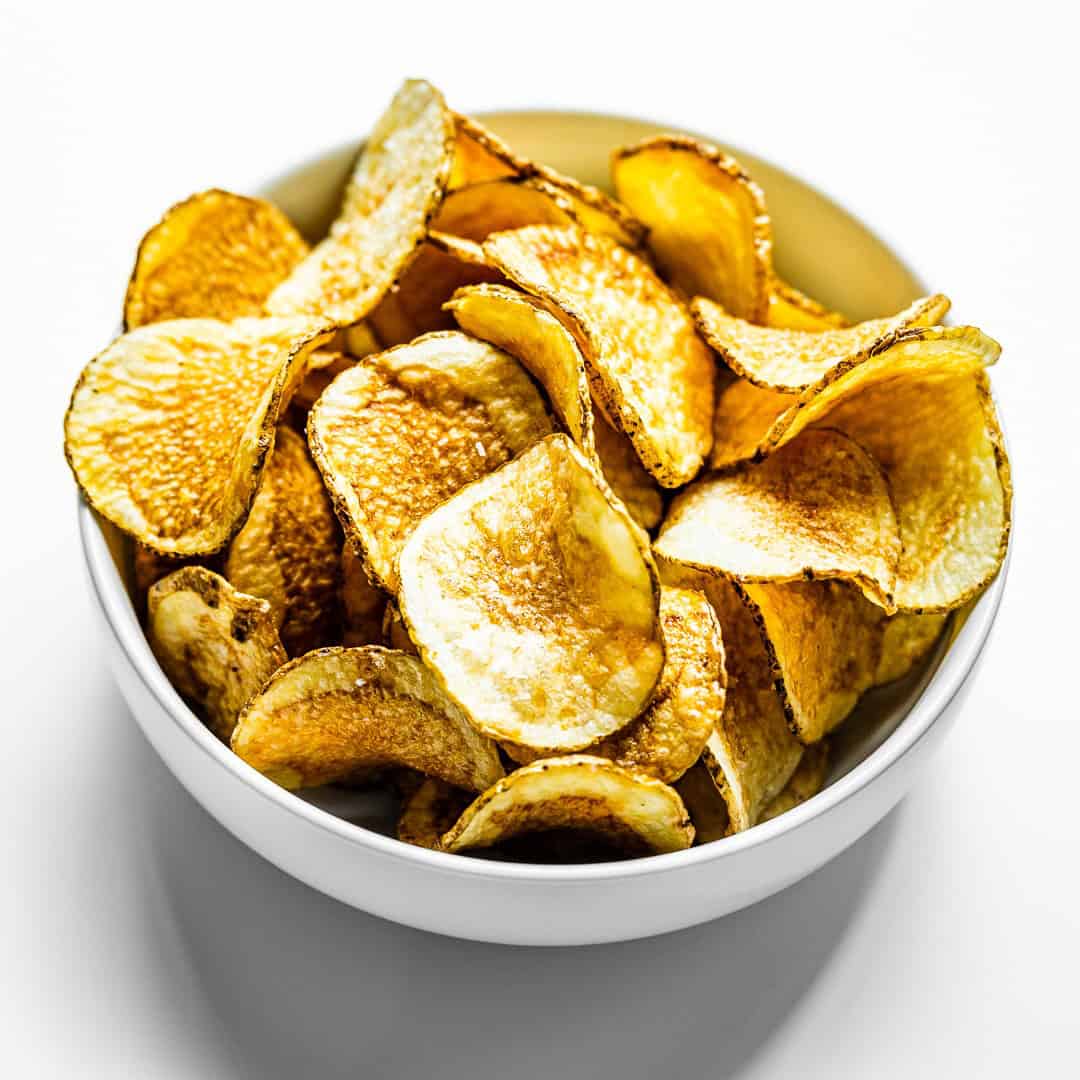This image features a white bowl brimming with golden-yellow potato chips, each chip presenting a slightly curved, Pringle-like arch. The chips appear handcrafted, as they retain the skins around their crispy edges, varying from a matte golden hue to darker, almost burnt-looking outlines, indicating they were either baked or fried. The bowl itself has a circular shape and a matte finish, sitting atop a white-grey background. The lighting highlights the chips, giving them a slightly reflective look, as if from a source above. The detailed texture and varied coloring suggest a homemade quality, making these chips an inviting snack, perfect for enjoying during a movie or a casual conversation with friends.